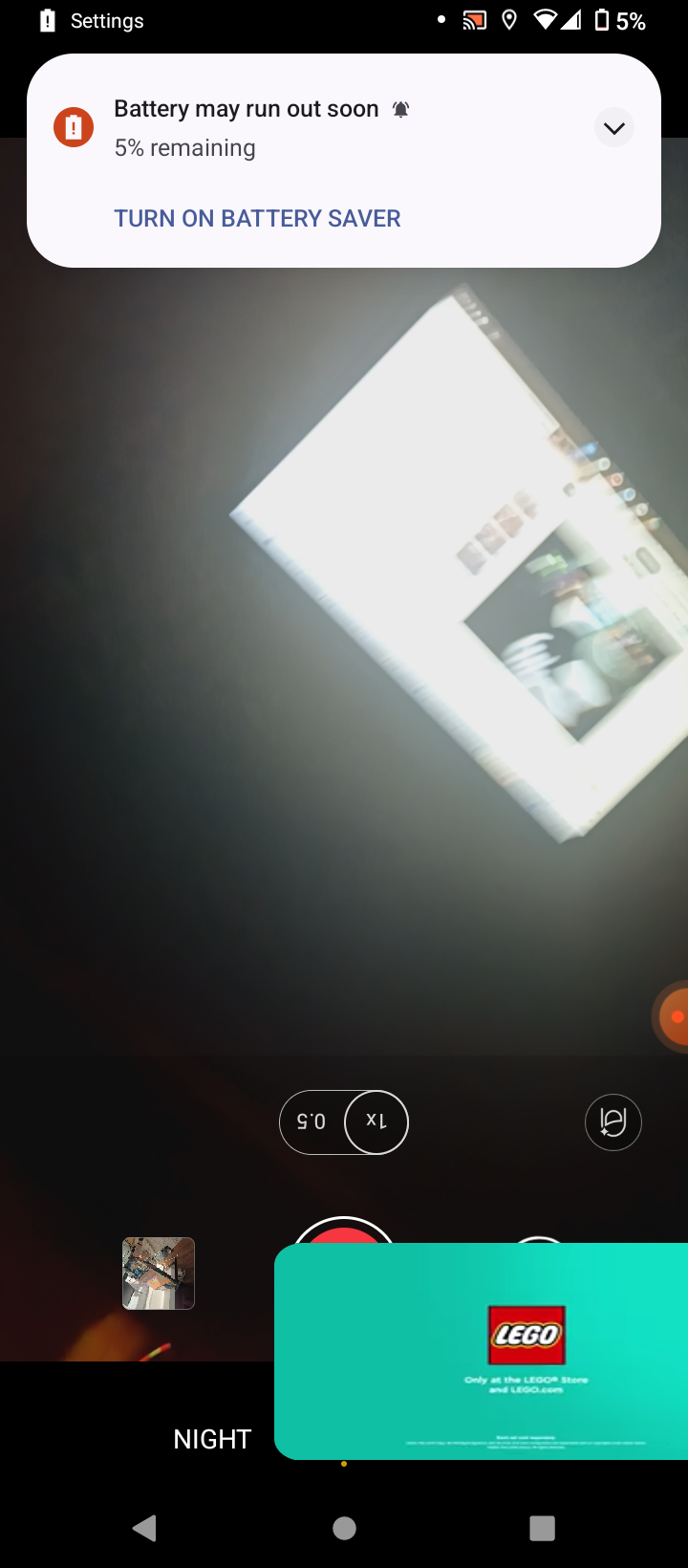This screenshot captures the moment a low battery warning appears on a smartphone screen.

At the very top of the screen, there's a typical status bar, which includes a battery icon with a black exclamation mark inside it, indicating an issue. To its right, the word "Settings" is displayed. Following an ample space gap, there is a white dot, presumably part of the interface design, followed by various icons: a screen cast icon in white and orange, location icon, internet connectivity icon, signal strength icon, and another battery icon showing 5% remaining.

Just below this status bar, a white rectangular pop-up with rounded corners appears, displaying an important warning in black text: "Battery may run out soon." Accompanying this message is a bell symbol and an orange circle holding a white battery icon with an exclamation mark, reiterating the critical battery level of 5%. The message also advises, "Turn on Battery Saver."

This alert overlays what appears to be the phone's camera interface. It shows a live view of the subject the phone camera was aimed at when the alert appeared. The view includes a bright white background emanating from a computer or TV screen, recognizable by the application bar at the top, suggesting the user was viewing a website.

Surrounding this brightly lit screen area, the environment is dark. The camera controls are evident at the bottom of the screen but upside down, displaying "1x" and "0.5x" options, and a large red button for capturing the image or starting a recording. Another notification, this one a blue rounded rectangle with the red Lego logo and some unreadable white text, is also visible on the screen.

Finally, at the bottom, the phone's navigation bar is shown, with an arrow pointing to the left, a circle, and a square symbol on the right. This bar partially covers the camera controls, but the word "Night" is still visible.

Overall, this screenshot poignantly captures the moment of a critical low battery alert interrupting the user while they are in the midst of taking a photo of a brightly lit computer screen.